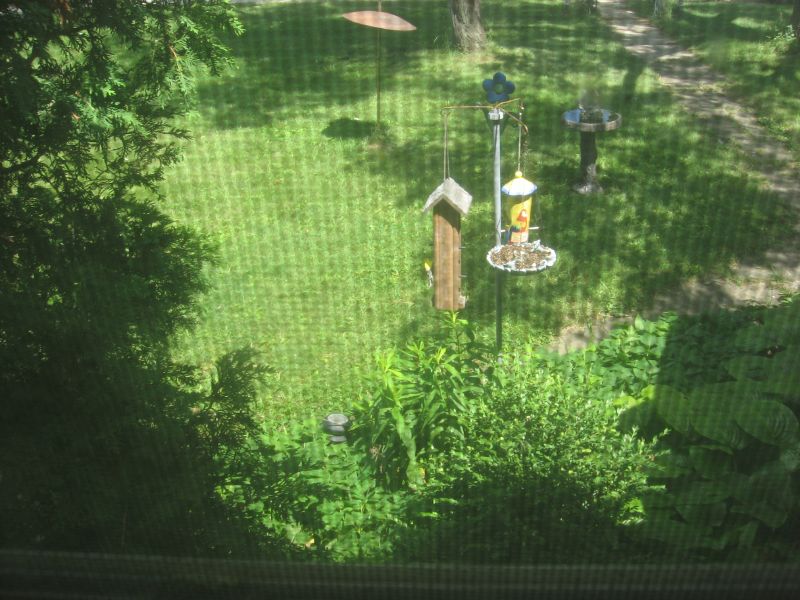The image depicts a serene backyard scene with several notable features. In the foreground, there's a wooden birdhouse with a whiteish-gray roof hanging from a rope attached to a metal pole that is adorned with a small, plastic green flower. A bird with a yellow head can be seen perched on the side of this birdhouse. Nearby, there's another birdhouse painted yellow, displaying an illustration of what appears to be a parrot. Below this birdhouse is a bowl filled with some kind of food. 

In the mid-ground, a birdbath, possibly made of black material, is visible to the right, and an umbrella stands to the left. Further back, a lush green lawn and a variety of trees create a tranquil backdrop. On the left side and bottom-left of the image, more trees can be seen, adding depth and richness to the scene. Additionally, in front of the camera, there is a screen that slightly obscures the view, indicating the photo might have been taken through a porch or window screen.